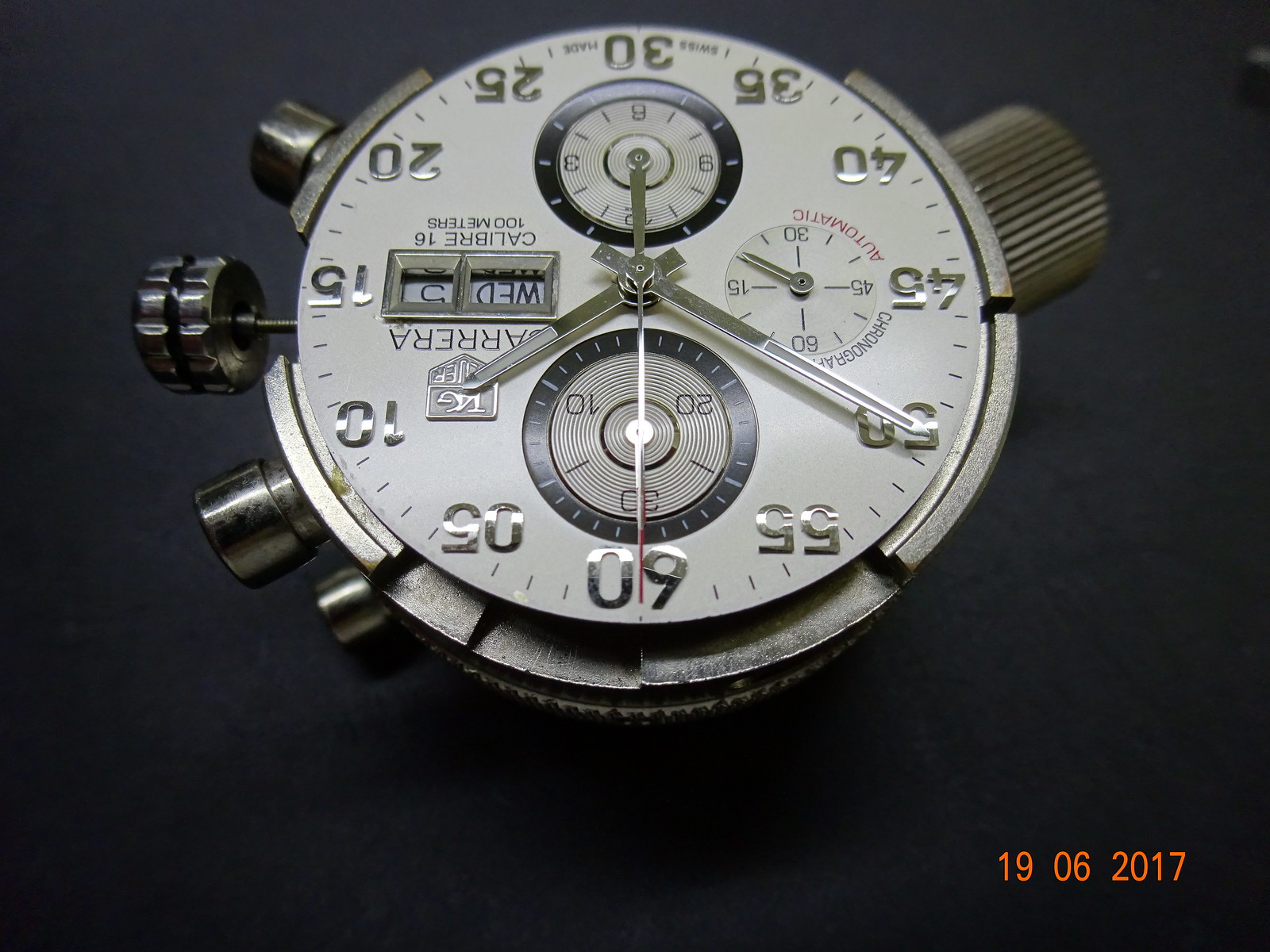This detailed close-up photograph showcases the face of a TAG Heuer watch, specifically the Carrera model, removed from its casing and placed against a solid black background. The watch face, creamy white in color with raised silver lettering, is positioned upside down in the image. Notable features include silver hands pointing to approximately the 10 to 2 position, and various dials and knobs visible on the sides. The face displays a sequence of numbers around the outer edge marking minutes in increments of five, from 0 to 60, with numerals like 05, 10, 15, 20, 25, 30 prominently noted. Additionally, the photograph reveals a chronograph feature on the right side (left when upright), which marks intervals up to 60. The current date, "Wednesday the 5th," appears alongside the TAG Heuer logo and "Carrera" inscription. Further markings include "19 06 2017," suggesting relevant dates or years associated with the timepiece. The photograph's perspective emphasizes the intricate details and craftsmanship of the watch.